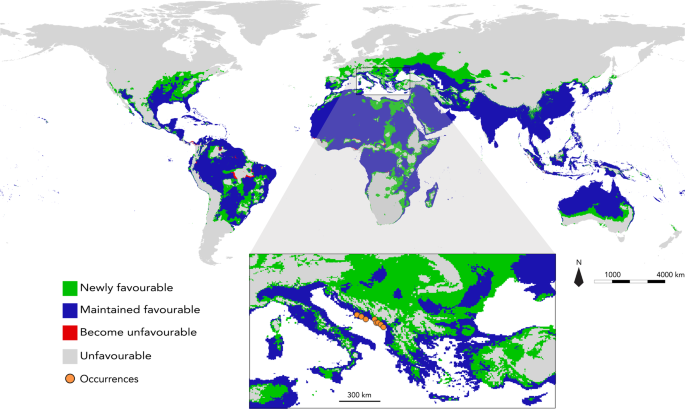This photo features a detailed world map with distinct color-coded regions, highlighting varying conditions across different landmasses. The map includes green, blue, red, and gray areas, each signifying different statuses: green indicates "newly favorable," blue shows "maintained favorable," red represents "become unfavorable," and gray denotes "unfavorable." Additionally, orange dots scattered throughout the map indicate specific occurrences. A key on the bottom left clarifies these color codes. The map primarily focuses on central global regions, with prominent blue and green areas across the middle sections, while the outer regions remain mostly gray. Specific zoomed-in areas, particularly around Europe and Italy, show detailed clusters of these color-coded regions and occurrences. The bottom right corner features a compass and a scale ranging from 1,000 to 4,000 kilometers, aiding in geographical orientation and distance measurement.